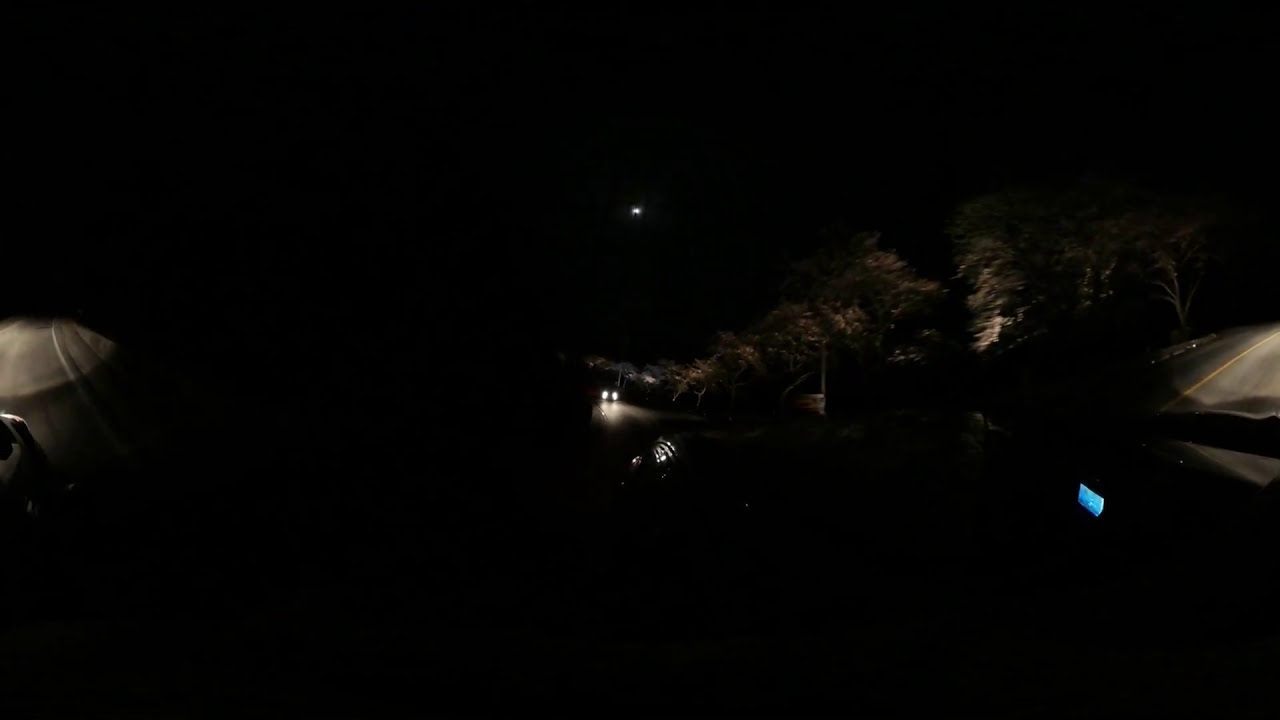This detailed nighttime panoramic image captures a moody, dimly-lit scene. Dominating the center is a dark roadway with a car traveling down the middle, its headlights casting a pair of bright beams onto the ground. To the top right of the frame, a cluster of trees can be discerned, illuminated faintly from below. The sides of the road, marked by yellow and white lines, stretch to the far left and right, reinforcing the panoramic nature of the photograph. The bottom right corner offers a glimpse into the vehicle’s interior, where cool blue lights from the dashboard are faintly glowing. High above the road, an isolated light in the black expanse might be the partially obscured moon, adding to the eerie atmosphere. The color palette mainly features deep blacks, interspersed with whites, grays, greens, oranges, tans, and yellows, highlighting the contrasting elements in this outdoor neighborhood scene in the heart of the night.